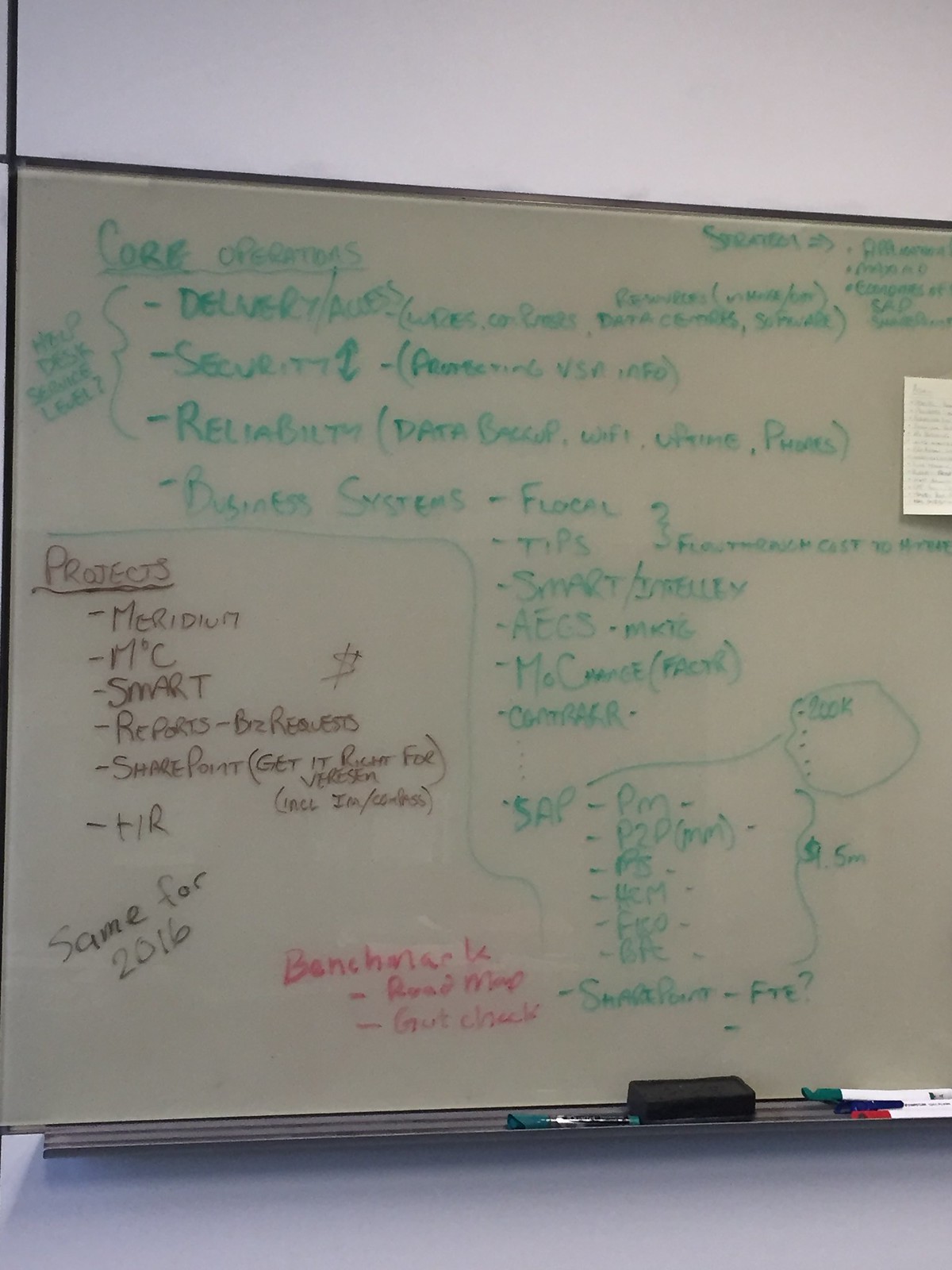This portrait-style image shows a classroom whiteboard with various notes and plans written in different colors of erasable ink. The whiteboard, mounted on a white wall and set against a light purplish background, captures approximately three-quarters of its length. 

At the bottom, the board is equipped with markers and a black eraser. The predominant writing is in green, outlining the "core operators" of an IT system, focusing on aspects such as delivery, security, reliability, and business support. This section appears to be an instructional or planning element, relevant to an IT help desk solution or similar project.

In brown ink, the whiteboard lists the names of specific projects, including Meridium, MC Smart Reports, Biz Requests, SharePoint, HR, indicating that these are likely for the year 2015, as referenced by a note in black stating "same for 2016." Red ink is used for benchmarks, adding another layer of planning details to the mapped-out IT project strategy. Additional terms like SAP and acronyms such as PM and PS further categorize the supported programs and project details, making this an organized yet intricate guide for IT initiatives.